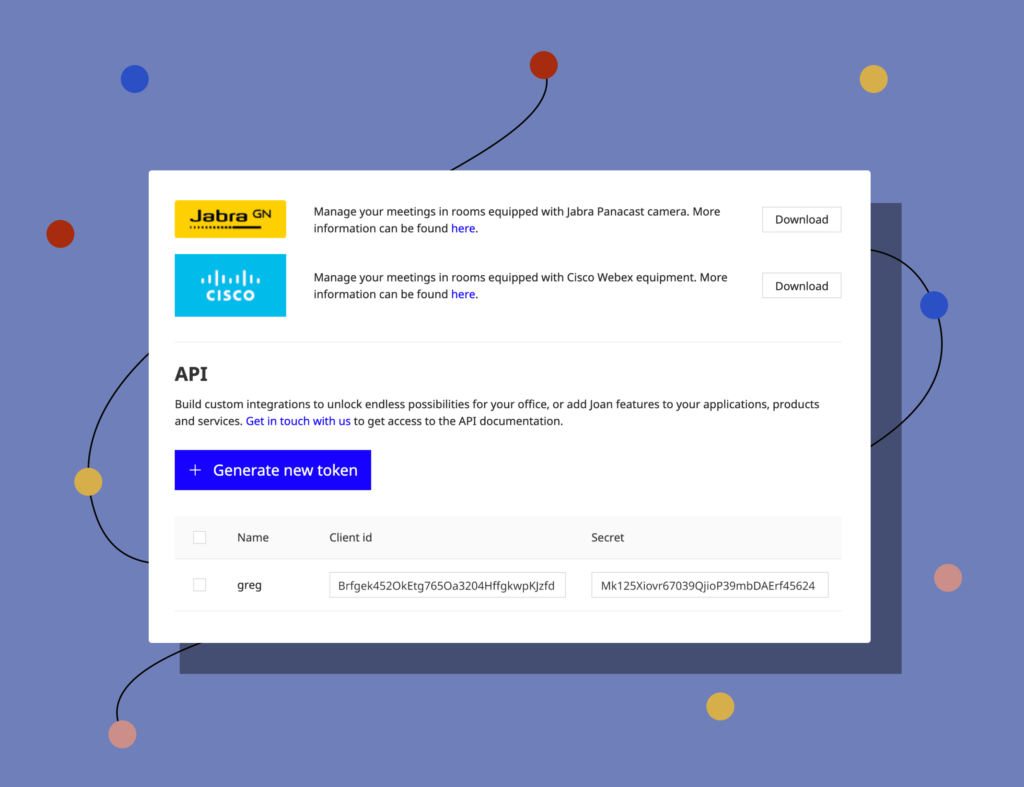The image features a background that is predominantly dark purple. At the center, a white rectangular tab is positioned equidistantly 2 inches from the top, bottom, and both sides. Surrounding this white tab in the purple backdrop are several colored dots and lines.

Starting from the upper area of the purple background, approximately 1 inch from the top edge, there is a blue dot. Directly below this, there is a red dot positioned at the midway point. To the right of the red dot, there is a yellow dot. A black line starts below the red dot, travels diagonally downwards to the left, and extends behind the white tab.

On the left side of the white tab, a red dot is situated, and further down towards the bottom, another yellow dot can be found. From this yellow dot, a black line extends leftwards and moves through it, disappearing beneath the white tab. This black line reemerges at the bottom left corner, connecting to a pink dot. On the right side of the image, towards the bottom, there is another yellow dot, positioned just above a pink dot. Additionally, at the top right, there is a blue dot with a black line that goes up and then down behind the white tab.

Inside the white tab:

- At the top left corner, within the white border, there is a yellow rectangle bearing the text "Jabra GN" in black letters.
- On the right side, there is a white rectangle with a gray border and black text that reads "download."
- Below the white rectangle, on the left side, is a blue square labeled "Cisco."
- Following the blue square, there are two lines of information and a download button again on the right side.
- Next, a thin, gray triple line appears, followed by the word "API" in bold, capitalized black letters.
- Beneath "API," two more lines of information are displayed.
- At the bottom, there is a blue tab with a white plus sign on the left side and the text "Generate New Token."
- Underneath this tab: 
  - "Name" is listed with a checkbox next to it.
  - Next to "Name," on the right, "Client ID" is displayed, followed by "Secret." Below each label, respective information is provided: "Name" says Greg, "Client ID" contains a unique identifier, and "Secret" holds the secret information.